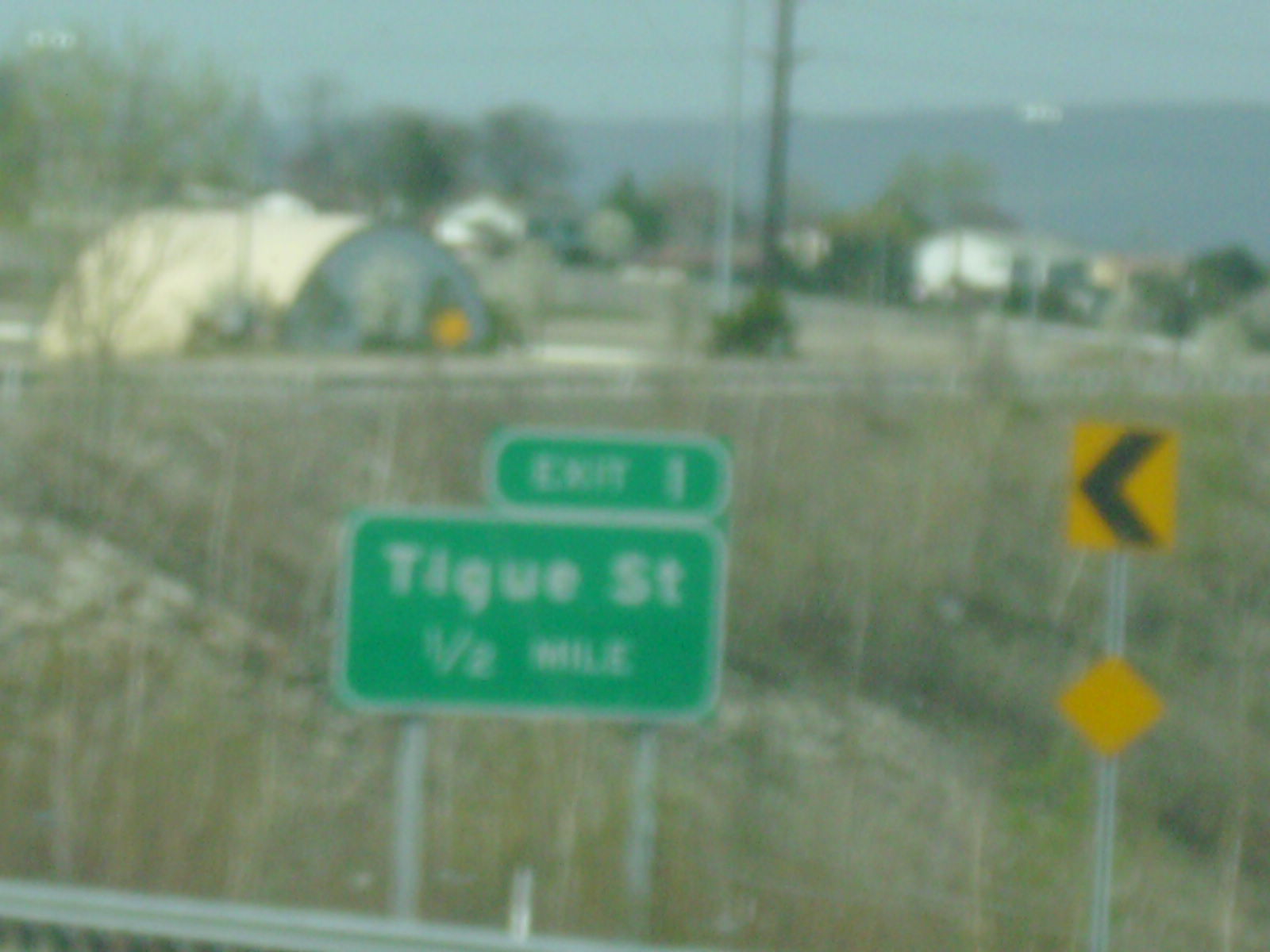The image captures a blurred scene taken from what appears to be a car window, showing a rural backdrop with fields and a domed-roof building. Dominating the foreground are two green highway signs: a smaller rectangular sign in the upper right corner reads "EXIT 1" in white, capital letters with a rounded white border, and a larger rectangular sign below it states "TIGUE ST, 1/2 MILE" in the same styling. No leaves are present, suggesting the image was taken out of season, though some greenery is visible amidst the sparse vegetation. To the right of these signs stands a tall yellow warning sign featuring a black left-turn arrow and a blank yellow diamond midway down the pole. The image also includes a silver guardrail at the bottom left and offers a view of pale green fields with trees in the background, under a grayish-blue sky merging with distant, darker mountains.